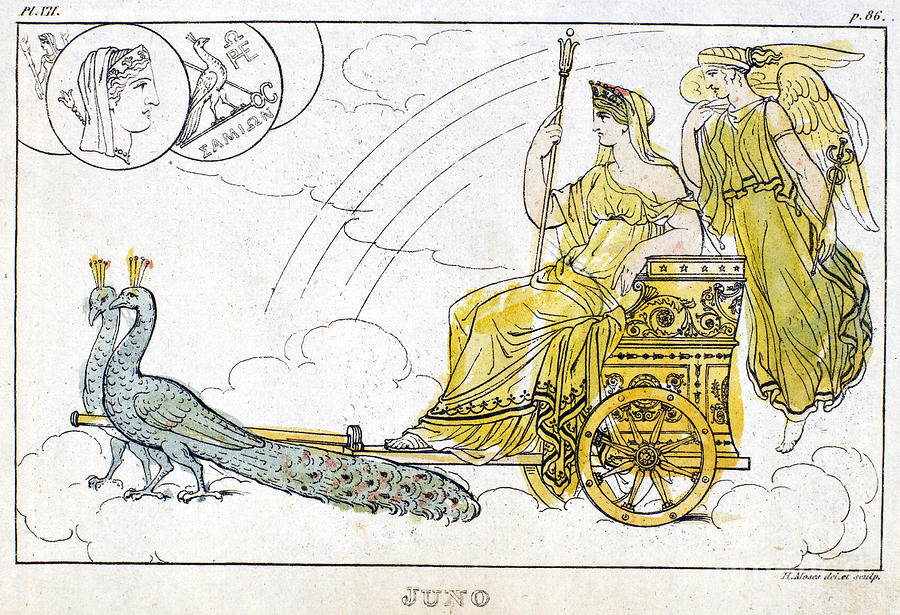This illustration, done in marker and resembling ancient Greek-style artwork, depicts an elaborate scene featuring two blue peacocks with vibrant highlights of orange, black, and red, pulling a beautifully ornate golden chariot. The peacocks, connected by a bar of steel, stand on what appears to be a cloud. The chariot, heavily engraved and detailed, houses a regal figure wearing sandals, a flowing golden robe, a golden shawl around the head, and a golden crown, holding a golden scepter topped with a small trident. Floating behind the chariot is an angel dressed in similar golden robes with striking golden wings, adding a celestial touch to this richly detailed and ethereal composition.